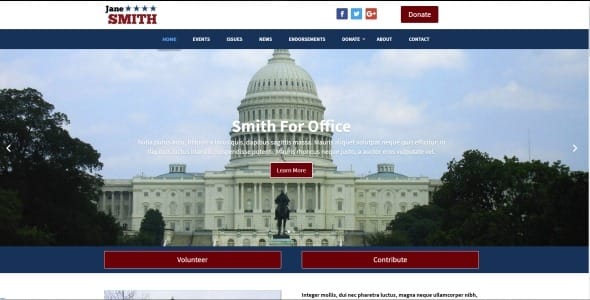The webpage features a clean white border and prominently displays the name "Jane **** Smith" at the top. To the right of her name, there are social media icons for Facebook, Twitter, and Google Plus. A conspicuous burgundy box labeled "Donate" is also present. Below this, a dark blue navigation menu spans the width of the page, including eight clickable options, though the text is too small and blurry to discern.

Centrally, a photo of the U.S. Capitol Building dominates the layout, flanked by trees and featuring a statue of an individual on horseback. Above the image is the campaign slogan "Smith for Office," accompanied by a block of text that's illegible due to its small size. 

Further down, a burgundy button labeled "Learn More" is prominently positioned. At the bottom of the page, two burgundy boxes are placed on the left and right sides; the left box reads "Volunteer," while the right one says "Contribute." The page rounds out with another image and some truncated text at the very end.